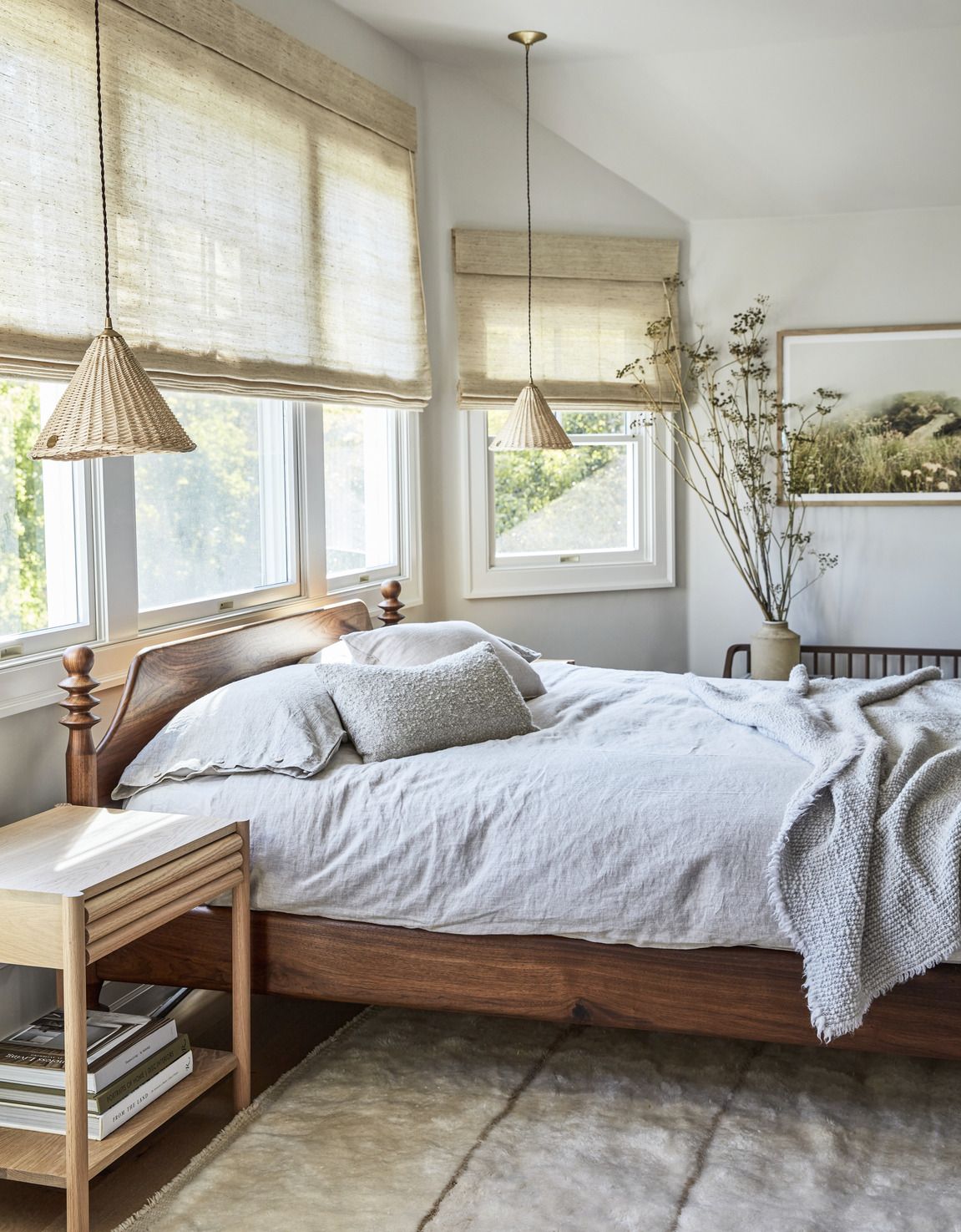The image captures a professionally staged, vertically rectangular full-color photograph of a bedroom, bathed in natural light. The walls are pristine white, matching the ceiling, and they frame the interior scene beautifully. Central to the picture is a large, short poster wooden bed, adorned with four white pillows and a matching white blanket. The bed rests atop a fluffy white rug, contributing to the room's airy and serene ambience.

Above the bed are three double-hung windows, each dressed with sheer, opaque gray shades that let in filtered light. Flanking the bed are two nightstands; the one on the left is light brown and includes some books on its bottom shelf. From the ceiling hang two pendant lights with basket-like wicker shades, casting a warm glow over the room.

On the far wall opposite the bed, a bench with railings houses a clay pot filled with tall branches or plants, adding a touch of nature to the interior. To the right of the bench, a framed picture displaying a serene landscape of trees and mountains hangs center-right on the wall. Just to the left of this artwork sits a planter, completing the room’s organic and welcoming design.